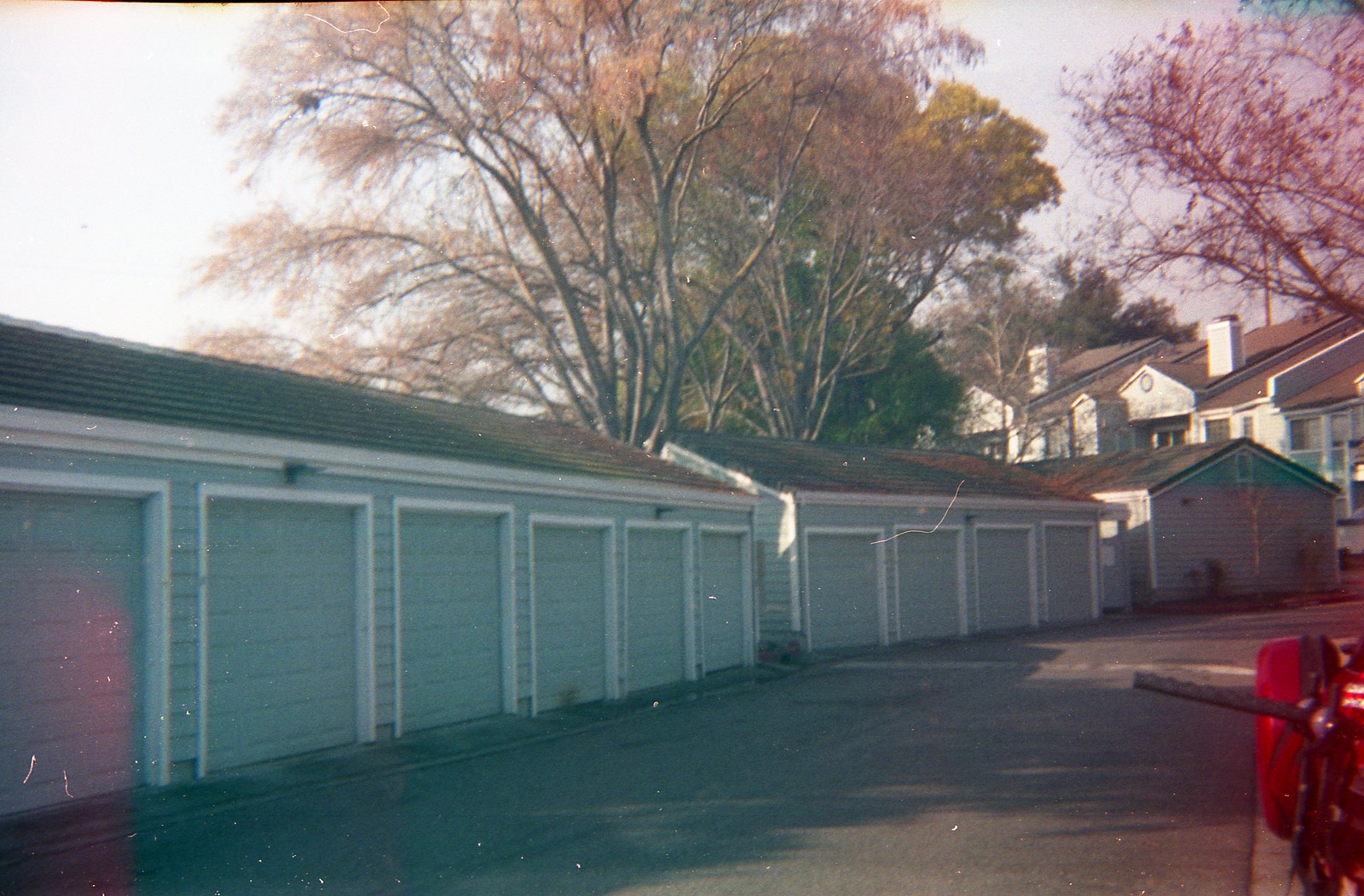The photo depicts a row of exterior garages, likely part of a condominium complex, featuring a total of ten garage doors spread across three interconnected buildings. These buildings are painted light blue with white trim and have brown roofs. The garages are situated on an asphalt surface with a road leading around the side towards what appear to be additional residential structures, potentially apartment complexes, following the same color scheme. In the background, large trees with a stunning array of yellow, green, orange, and reddish leaves tower over the garages, offering a vibrant contrast. The sky is a bright white, indicating a sunny day with visible shadows cast in front of the garage doors. In the bottom right corner, there's an object with red and white stripes, possibly a pole with a holder.